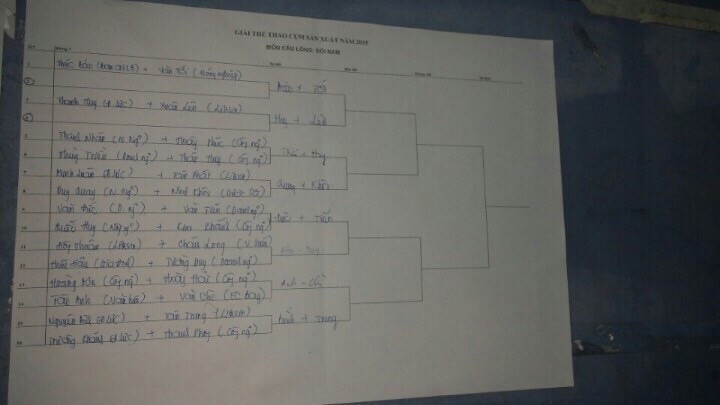The image depicts a low-quality, blurry photograph of a large white piece of paper attached to a blue wall or background indoors. The paper, which is wider than it is tall, features a printed bracket commonly used in tournaments. At the top of the paper, two lines of black text serve as a header, although they are illegible due to the photograph's poor quality. The bracket shows a layout of several rounds, with lines and numbers indicating progression from left to right. The first stage is populated with the names of 14 teams or groups, but two slots are blank, possibly indicating forfeits. Blue ink is used to fill in the teams' progression, with the second stage showing 8 remaining contenders. The bracket appears to progress through four rounds, culminating in a final fifth stage for the champion. The numbers "1 to 7" are listed on the left side, aligning vertically, likely denoting stages or rankings within the bracket. Overall, despite the image's low resolution and darkness, it clearly presents a tournament's structured progression.